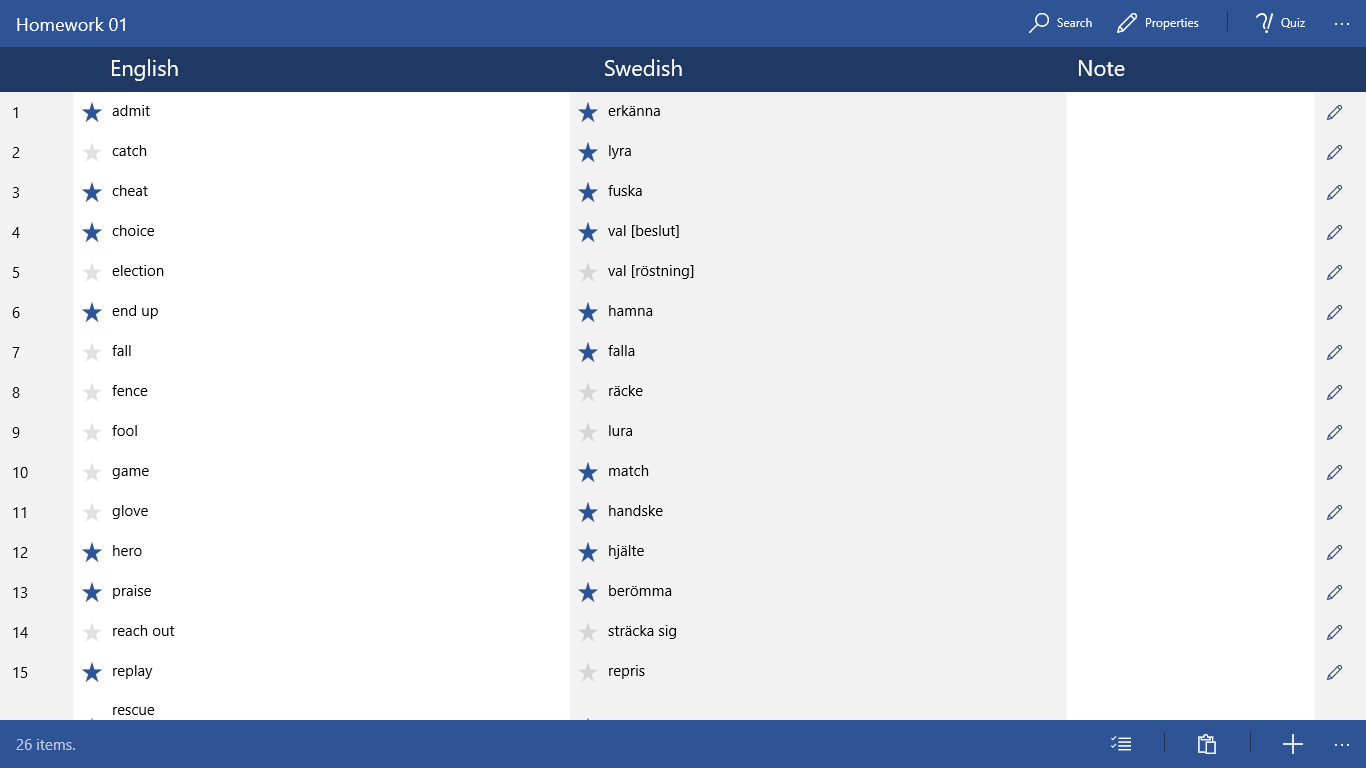The image captioned "Homework 01" displays a detailed layout with a blue background and black text. In the top right corner, white text labels several options: "search," "properties," and "quiz." Below the header, the background shifts to a darker blue, organizing information into three columns labeled "English," "Swedish," and "Note." The Note column remains empty. The main content area features a white background.

Under the English column, items are listed with numbers from 1 to 15, alongside stars indicating their selection status. Selected items are marked with blue stars and include the words: "admit," "choice," "cheat," "hero," "paradise," "praise," and "replay." Non-selected words, indicated by grey stars, include "catch," "fall," "fence," "fool," "game," "glove," "reach out," and "rescue."

The Swedish column mirrors the English column, with selected items such as "Ekana," "Ira," "Fuska," "Val," "Beslat," "Hamna," "Fala," "Match," "Henske," "Hajle," and "Paroma." Non-selected terms include "Val," "Rosning," "Rake," "Lura," "Trakassic," and "Reprise." 

The bottom left corner of the image notes the total count: "26 items."